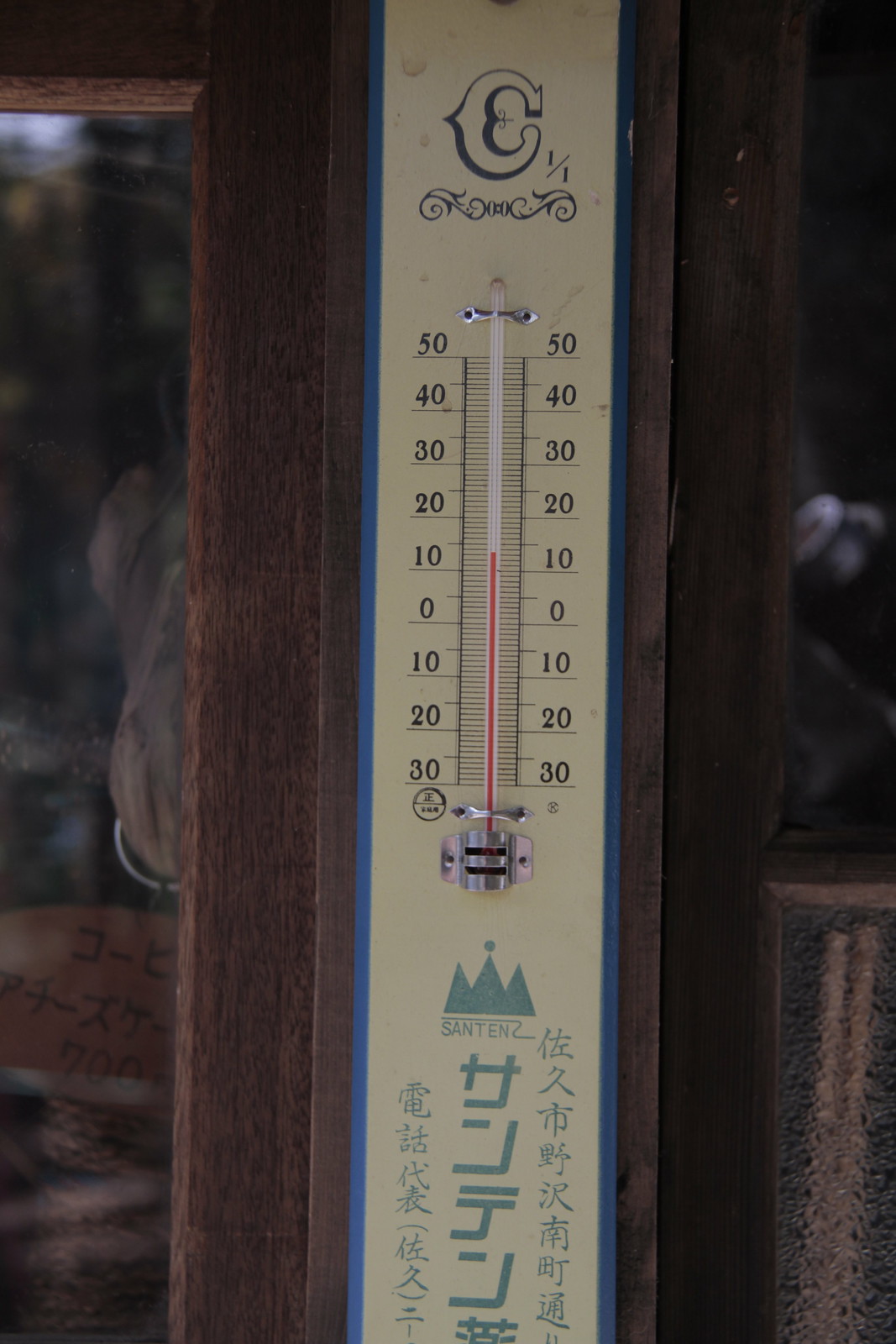A Celsius thermometer with Japanese or Chinese writing is mounted against a tan background. The thermometer features a distinct design with three peaks, the middle peak marked by a dot, and the text "San 10" displayed prominently. The black lettering contrasts sharply with the background, enhancing readability. It reads approximately 14 degrees Celsius, indicating a cold environment. The thermometer is encased within a blue border and is attached to a wooden frame, possibly part of a door or window. Glass panels are visible on either side, suggesting it could be the mullion where two window frames meet. The exact location, indoors or outdoors, remains uncertain.